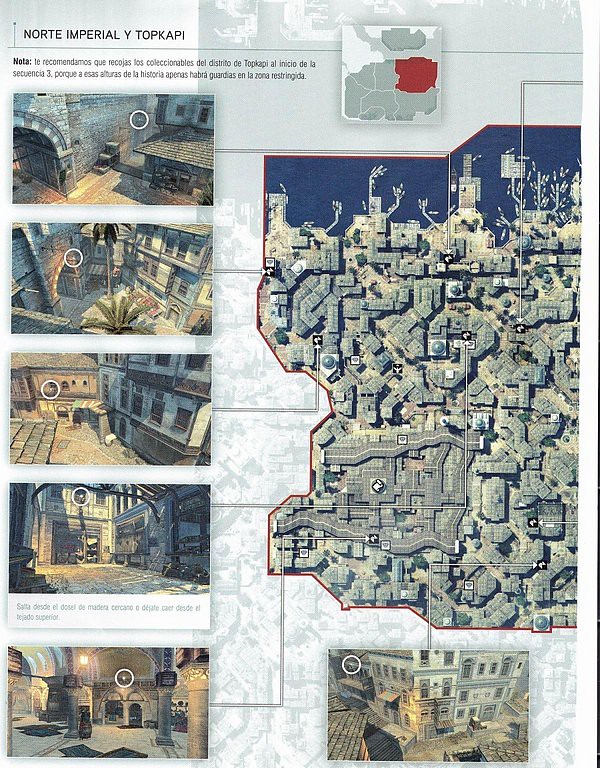This image depicts a detailed, overhead look at a vintage-style map likely from a video game. The map, set against a gray background, is titled "Norte Imperial Y Topkapi" in black lettering at the top and along the left side, followed by two smaller sentences of black text that are too small to decipher.

Along the left side of the page, there are five inset illustrations showcasing various parts of a coastal city. These include views of rooftops, the side of a building adorned with a palm tree, a street-level scene with the city's skyline in the background, a narrow alleyway, and an interior of a building featuring a person. These illustrations exhibit a quaint, possibly historical urban layout, with stone walls, archways, gates, and various houses.

On the right side of the page, there's an overhead map of the entire area, outlined in red. The top quarter of this map displays blue water, suggesting a coastal port area with docks, while below it are various squares representing roads and buildings. At the bottom right corner, there is another inset illustration showing a different segment of the city.

Superimposed over the entire composition is a faint, larger grayscale map, adding to the vintage, historical ambiance of the presentation.